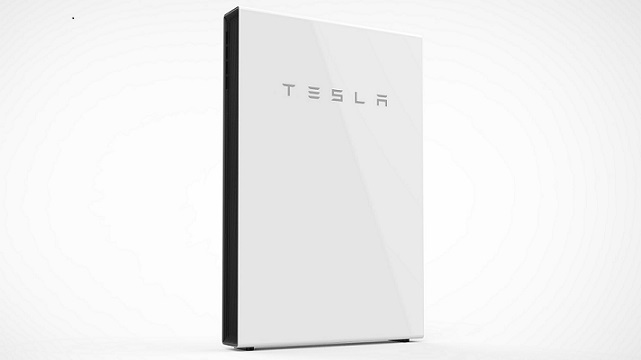The image portrays a rectangular object that is approximately twice as wide as it is tall, composed of subtly varying shades of gray. The periphery of the rectangle, particularly the corners, appear slightly darker, while the central area brightens to an almost white hue. Intricate lines emanate from the center towards the edges, reminiscent of tree rings or gentle waves.

At the heart of the image, a form resembling an open book is visible. The left side of this book-like shape, which mimics a spine, is positioned slightly closer than the right side and is distinctly black in color. The front cover of this 'book' is predominantly a light gray to white gradient.

Approximately two inches from the top edge and centered an inch from both the left and right sides, the word "Tesla" is prominently featured on the front cover. The logo is stylized; the "E" lacks the middle horizontal line, and the "A" is depicted as an inverted "U" with a line over it. 

In addition to the shadowing below the title, diminutive black feet are discernible on both the left and right sides, adding to the three-dimensional illusion of the object.